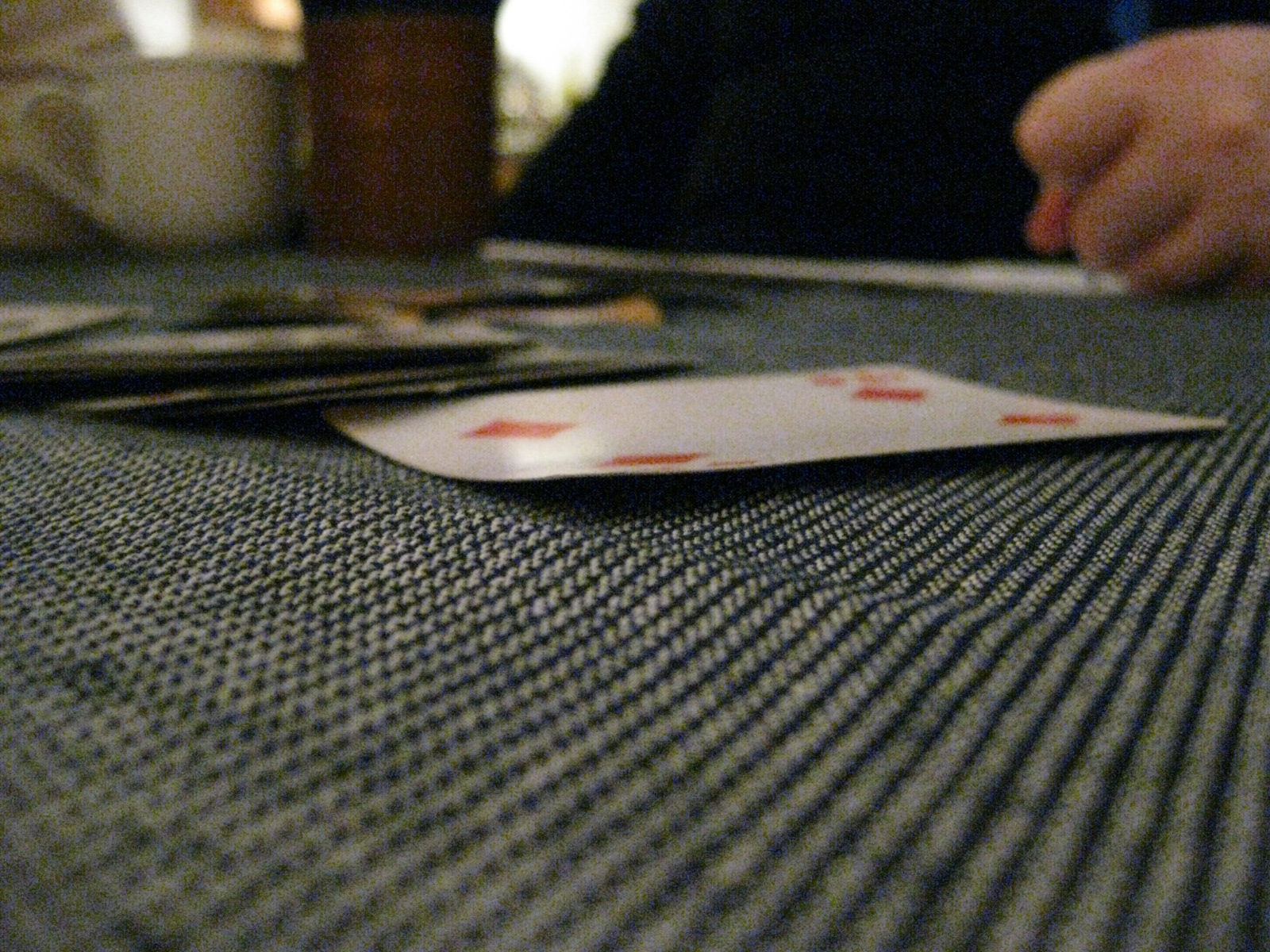In the image, a deck of playing cards is spread out on a flat surface, with the cards facing up. The only clearly visible card is the Four of Diamonds, which is white and prominently features four red diamond symbols arranged centrally, along with the number "4" in the top left and bottom right corners. The surface beneath the cards is a textured mat, blending shades of brown, black, and blue. 

Towards the far end of the table, a white mug and a brown cup are positioned. On the opposite side, a male figure is seated, partially visible. He is wearing a black shirt with a small blue emblem or color detail in the center. His right hand, appearing light-skinned, is placed on the table in a fist-like position, showing three covered fingers and a visible thumb.

Adjacent to the man, there's an object that might be a magazine or a phone; it is predominantly black with some yellow elements. The overall scene suggests a casual and relaxed environment, possibly during a break or a leisurely activity.